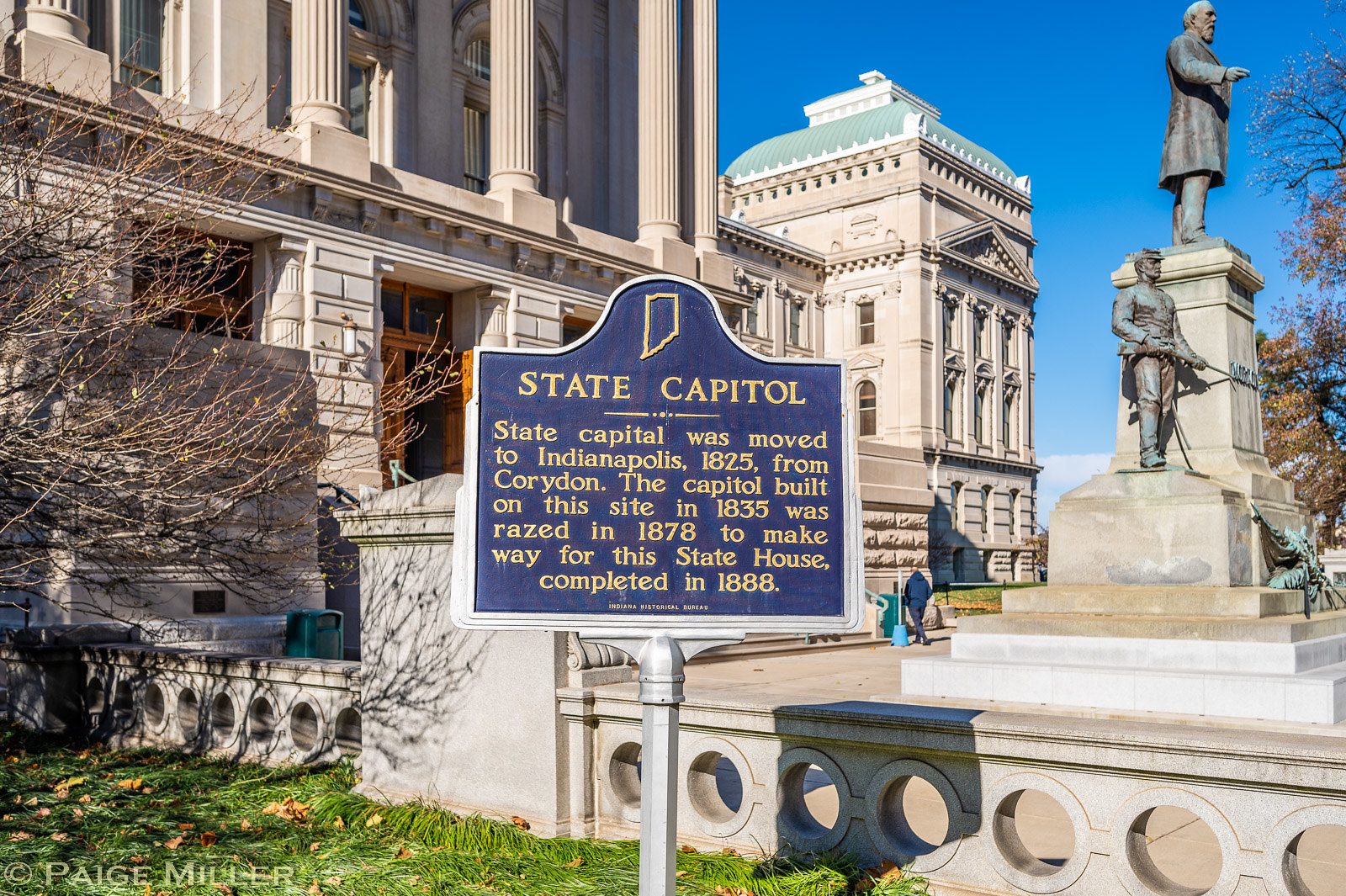This photograph features a majestic, light brown building with Roman-style pillars, known as the Indiana State Capitol. The building, constructed in 1888, stands tall with numerous columns and is adorned with statues—one depicting a soldier with a gun and another of a man atop a larger column gazing into the distance. In front of this imposing structure is a meticulously maintained garden area with lush green grass. Prominently displayed in the foreground center is a blue sign with raised yellow lettering on a silver pole and bordered in silver. The sign reads: "State Capitol. State Capitol was moved to Indianapolis 1825 from Corydon. The Capitol built on this site in 1835 was razed in 1878 to make way for this State House completed in 1888." At the top of the sign is an illustration of the state of Indiana. Surrounding the scene are some trees, and the sky is clear, adding to the grandeur and historic significance of the site.